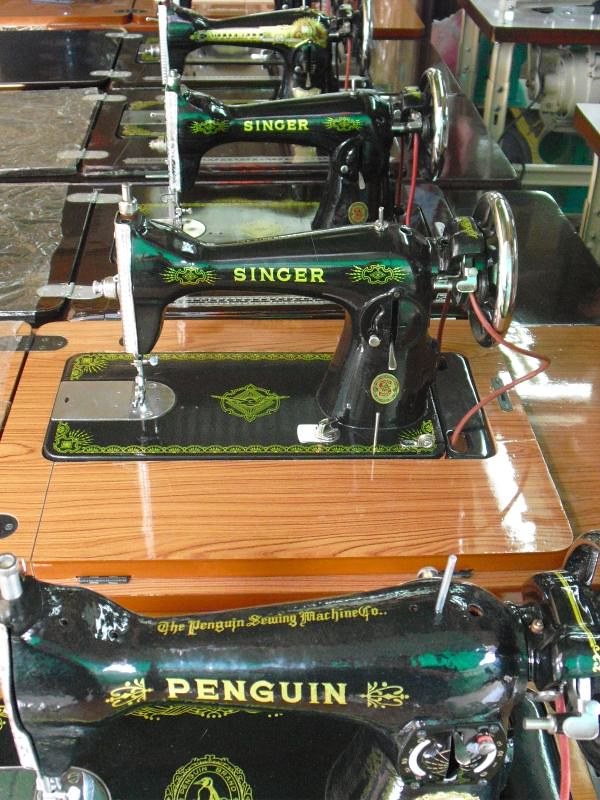The image depicts an antique shop showcasing a row of five antique sewing machines, prominently featuring brands like Singer and Penguin. Each sewing machine is elevated from its sewing machine cabinet, revealing their intricate designs. Four machines are set in dark wooden tables, while one rests on a lighter oak-colored table. The sewing machines are primarily black, adorned with decorative golden trim, and they display models and brand names in lime green and gold accents. The closest machine to the camera is a Penguin sewing machine with a detailed gold logo of the Penguin Sewing Machine Company on top. Positioned next are two identical Singer machines, marked by the yellow-green "SINGER" lettering and matching green star patterns. The final machine at the far end also features elaborate gold design work along its side, though the brand name is obscured. Each machine's functional elements, like the metal needle plate, side wheel, and red wiring, are also visible, showcasing their vintage craftsmanship.